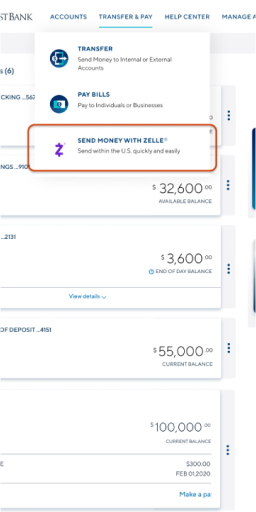In this image, we observe a section of a bank’s online interface, specifically highlighting the "Transfer & Pay" section. At the top of the screen are navigation tabs with "Transfer & Pay" prominently selected, flanked by other tabs labeled "Accounts" to the left and "Bank" adjacent. The focused "Transfer & Pay" section features options to "Transfer," "Pay Bills," and "Send money with Zelle," the latter being distinctly marked with a red outline, indicating an active selection for sending money via Zelle.

On the left side of the screen, there's a "Help Center" button, while the right side displays a "Manage" button. Below these, various account balances are listed, including figures such as an available balance of $32,600, an end-of-day balance of $3,600, a current balance of $55,000, and another current balance of $100,000. The bottom part of the image shows a partially visible button that begins with the word "Make," suggesting clickable functionality for a specific action, likely related to account management or transactions.

The provided directions and highlighted options imply that the image serves as a guide for transferring money using Zelle within the bank’s online platform. Overall, the interface illustrates different account balances and selected actions, offering a snapshot of the bank’s digital banking features.